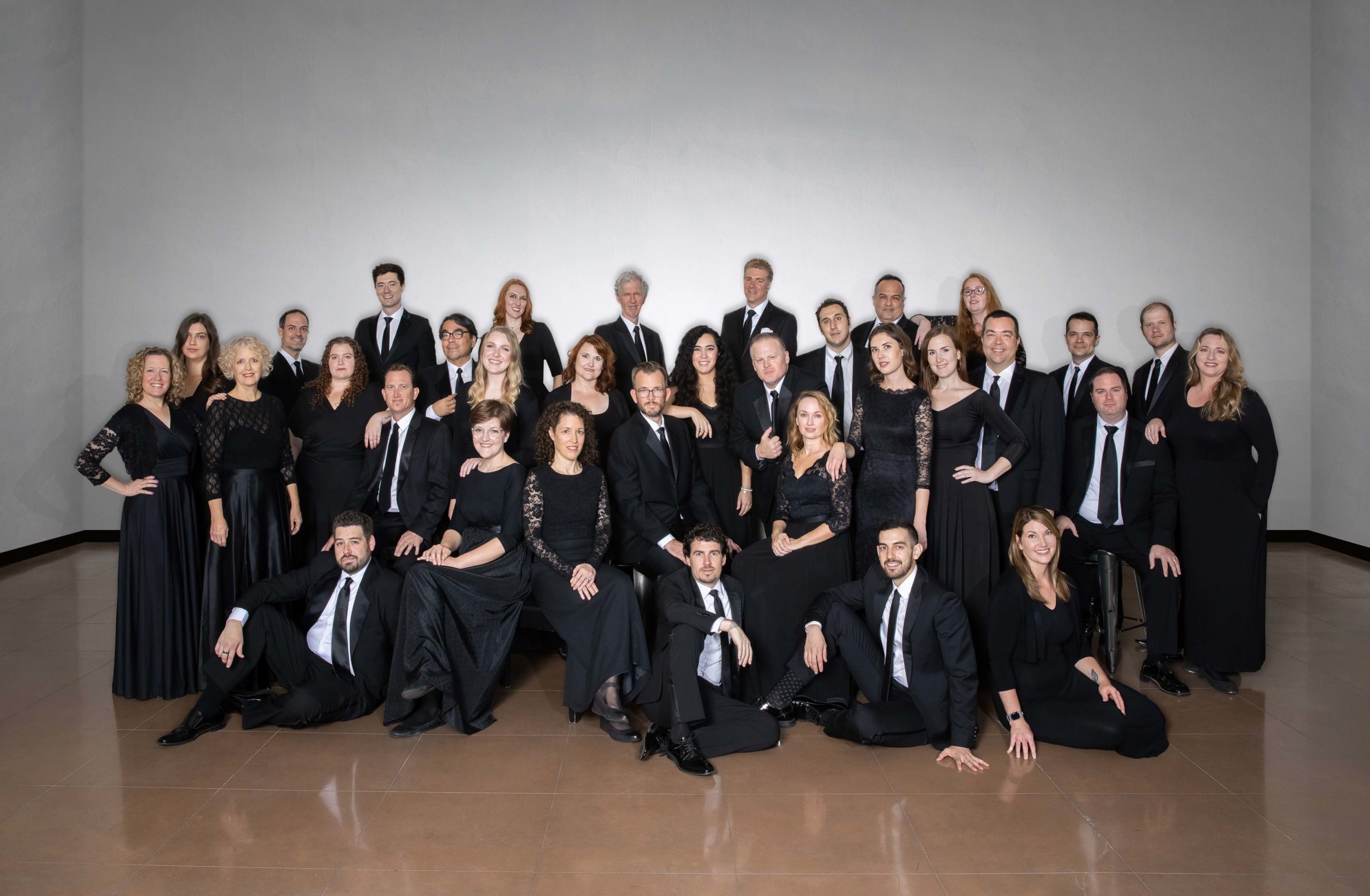This color photograph captures a large, formal gathering of around 30 Caucasian men and women, presumably performers, posed in a theater-like setting with light gray, white backdrop and a shiny, possibly marble floor. The attendees are elegantly dressed; men in black suits, white shirts, and black ties, and women in long black dresses, some featuring lace detailing. They are arranged in a meticulously organized formation: three standing rows at the back, a seated row on chairs, and four individuals sitting on the floor in the front. Despite their elegant attire, there are no visible instruments, suggesting they might be singers. The clean white walls behind them add to the formality of the occasion, and most individuals have pleasant smiles, enhancing the photograph's warm, collective atmosphere.